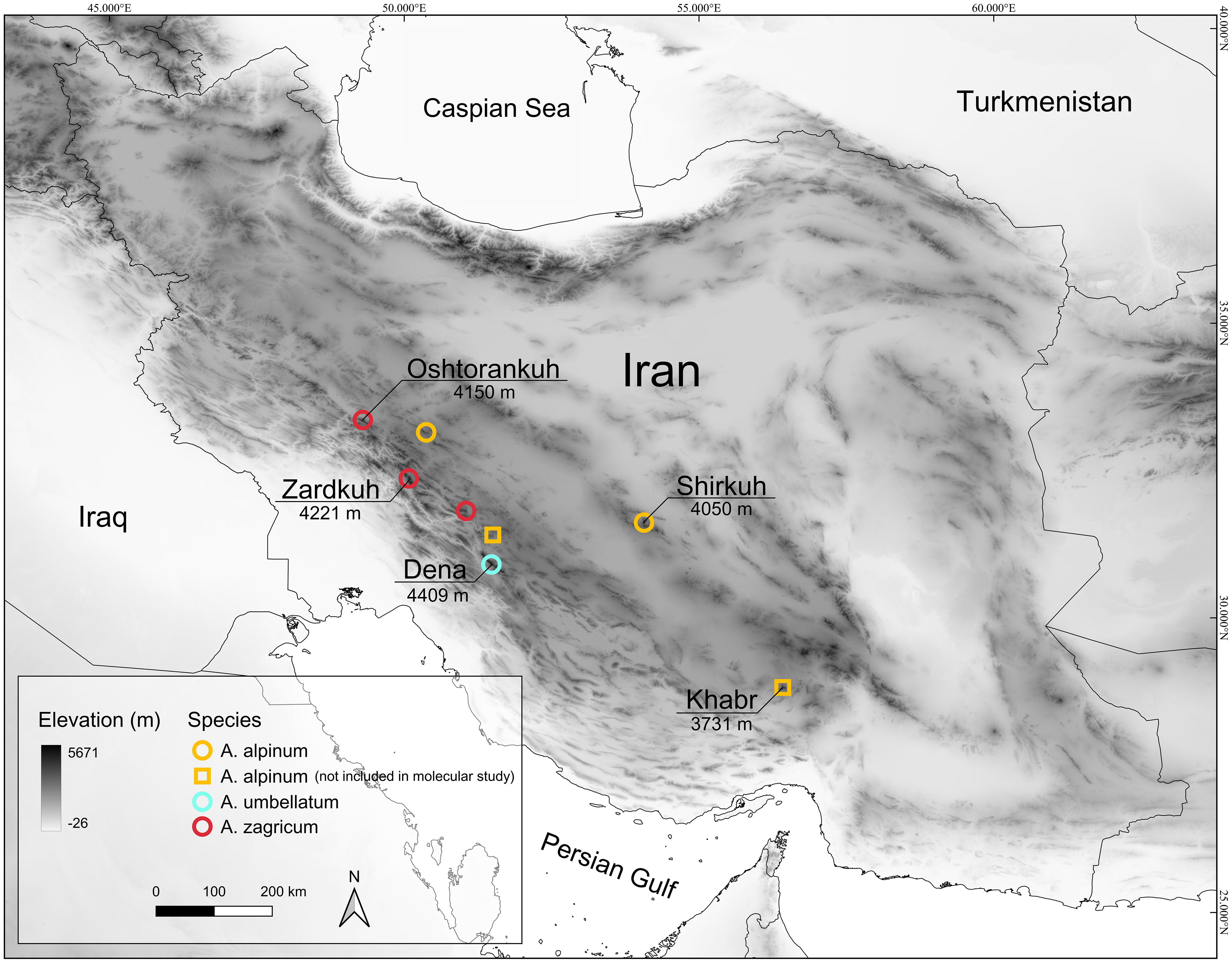This detailed, black, gray, and white map depicts a region of the Middle East, showcasing countries such as Iran, Iraq, Turkmenistan, and significant water bodies including the Caspian Sea in the upper part of the image and the Persian Gulf at the bottom center. The map displays varying elevations, with darker shades indicating higher altitudes ranging from 28 to 5,671 meters, as illustrated by the elevation legend. Several towns and cities across the mapped area are marked with colored circles and squares: yellow circles represent A. alpinum, yellow squares denote A. alpinum not included in molecular study, teal circles signify A. umbilicum, and red circles indicate A. zagiricum. These locations correspond to different species, as specified in the key located in the lower left-hand corner of the map. The map also includes a distance legend, showing measurements in kilometers, and an arrow indicating Compass North. Highlighted cities include Kabar, Shirku, Ashtoranku, and Zardku, with these colored markers helping to identify geographic and species distribution in the region.